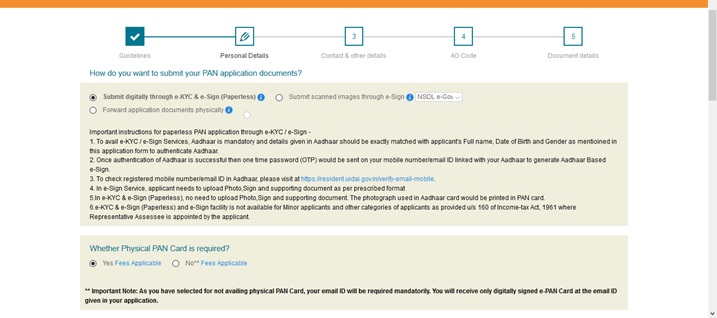The image is a low-resolution screenshot displaying a partially visible section of the PAN application page. Starting from the top, the screenshot shows several checkboxes arranged in a horizontal sequence. The first checkbox, labeled "Guidelines," is checked, suggesting the user has read or acknowledged the guidelines. Adjacent to it is a checkbox with an icon resembling a pencil or pen, labeled "Personal Details," indicating the current step the user is possibly working on. The subsequent checkboxes are labeled in sequence: "Contact and Other Details" marked as step 3, "AO Code," and "Document Details."

Beneath these checkboxes, a segment prompts the user with the question: "How do you want to submit your PAN application documents?" This is followed by options that the user can select, accompanied by crucial instructions for a paperless PAN application.

Further down, there is an area where the user can indicate whether a physical PAN card is required, with selectable options for 'Yes' or 'No.'

The overall background of the screenshot is white, and to the far right, the image captures the outline of a scroll bar with the bottom arrow visible, suggesting that the page has more information below what is visible in this partial view. The presence of the scroll bar indicates that this is a partially visible capture of the entire PAN application interface.